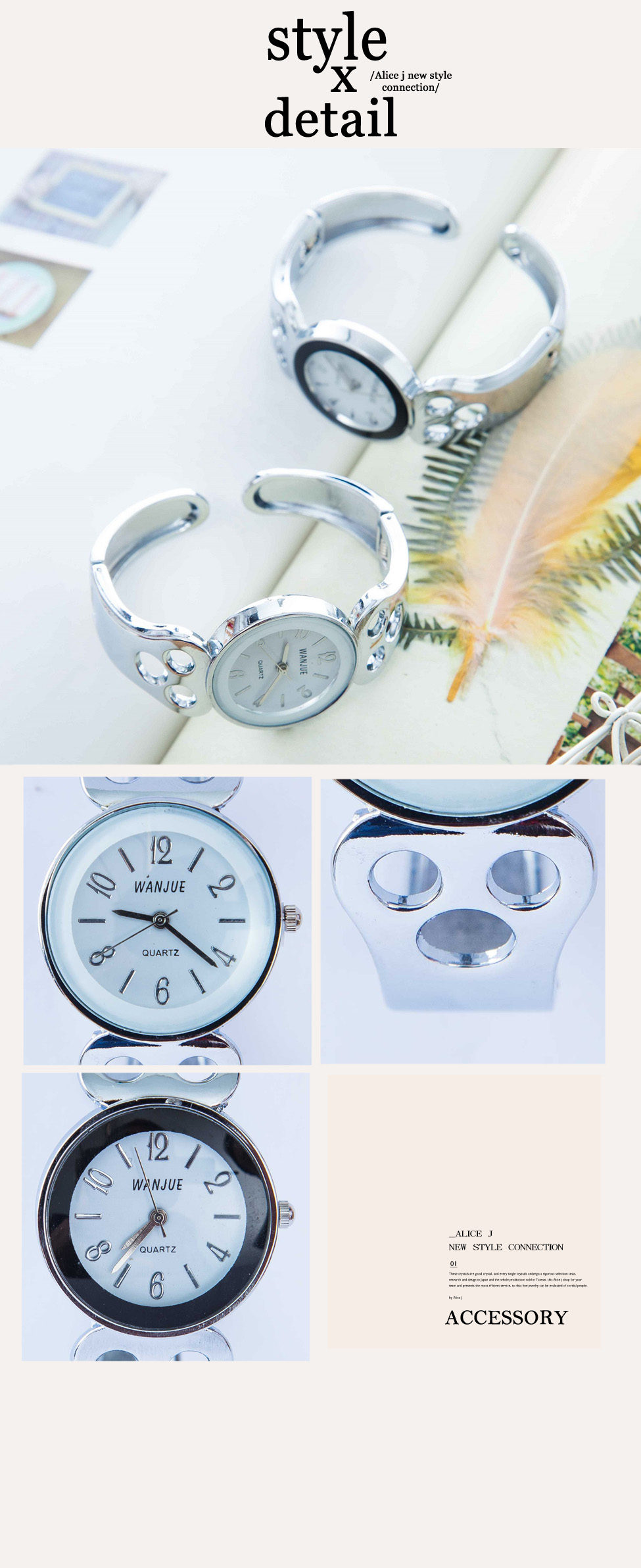This image features a beige background adorned with four photographs of elegant wristwatches. The top photograph showcases two silver wristwatches artfully displayed on a light-colored surface. Below this, closer shots capture intricate details: one highlights the watch face, while the other zooms in on the watch band, showcasing its craftsmanship. Overarching text along the top reads "Style X Detail" in bold black lettering, while the word "Accessories" is prominently displayed at the bottom. Additional text is present but too small to discern. This layout and imagery suggest a refined focus on timepieces, emphasizing both style and intricate detail.